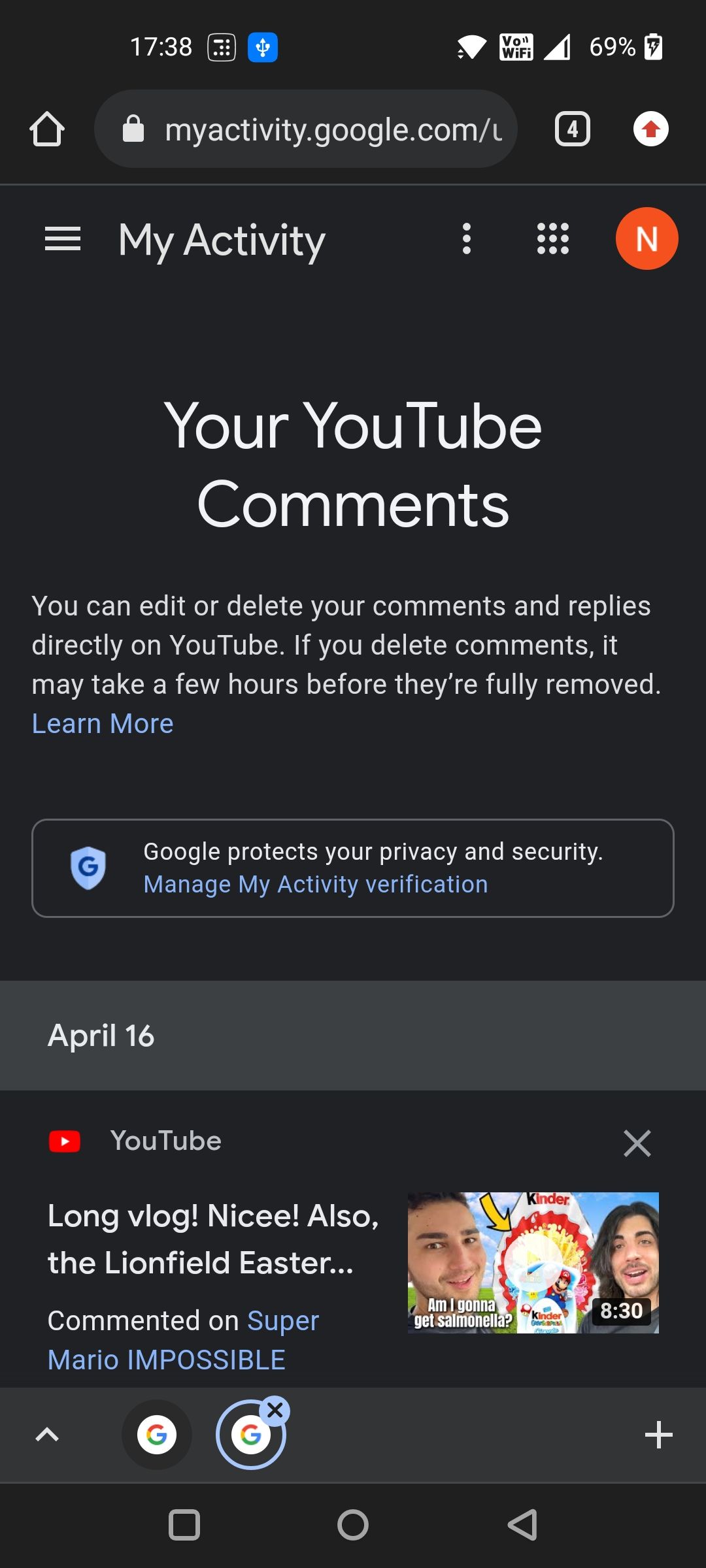The image displays a phone screen, with the time shown as 17:38 and the battery at 69% along with a Wi-Fi signal icon. The screen is on the "myactivity.google.com" page under the section "Your YouTube Comments." It states: "You can edit or delete your comments and replies directly on YouTube. If you delete comments, it may take a few hours before they are fully removed. Learn more." There's further information about Google protecting user privacy and security, alongside the option "Manage My Activity Verification." 

Dated April 16th, the screen shows specific YouTube activity, including a comment with the YouTube logo marked by an 'X' beside it. The comment reads "long vlog nice!" with an exclamation point. Another comment by "Lionfield Easter" mentions "commented on Super Mario Impossible." 

To the right, a thumbnail of a YouTube video is visible, featuring two men with sunny skies and green grass in the background. Between them is a Kinder candy bar pointed at by a yellow arrow. Overlaid on the image in white print are the words "Am I going to get salmonella?" The video has a timer at 8 minutes and 30 seconds.